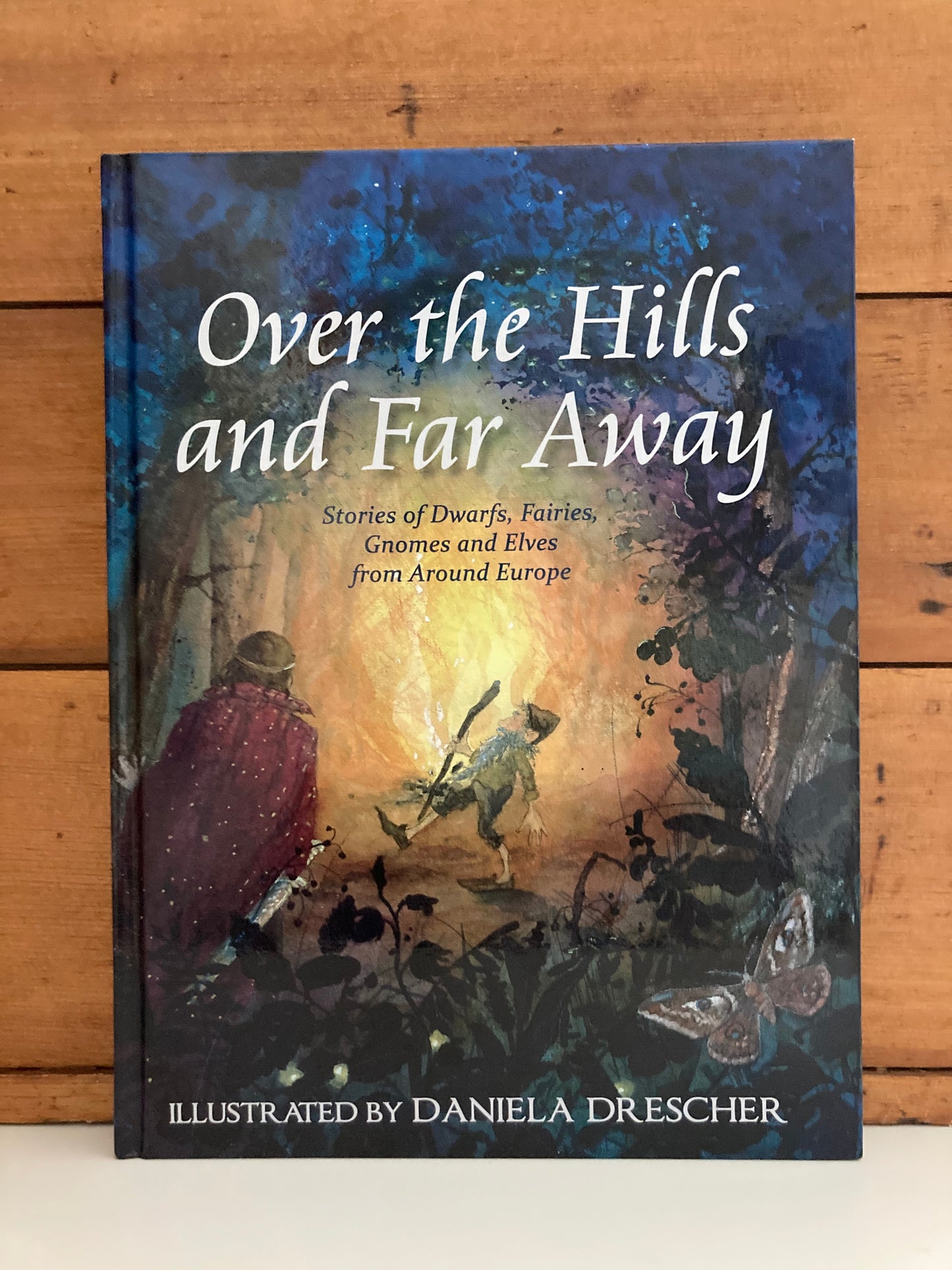The image depicts the cover of a children's book titled "Over the Hills and Far Away." The title is elegantly written in white script font across the top. Beneath the title, in black text, it reads: "Stories of Dwarfs, Fairies, Gnomes, and Elves from Around Europe." At the bottom of the cover, it is marked "Illustrated by Daniela Drescher." The hardback book features a blue background with an enchanting scene set at night in a dark forest. An ethereal light illuminates the center, where a gnome-like figure holding a walking cane appears to be stomping angrily. To the left, partially visible is a person, likely a woman, dressed in maroon clothing and a cape, appearing to watch the gnome. The lower part of the cover is adorned with brush and plants, framing the central scene. Adding a touch of whimsy, a butterfly flutters at the bottom right corner. The entire cover is a painting, rich with fairy tale elements that capture the magic and mystery of European folklore. The book lies against a wooden paneled wall, resting on a white floor.